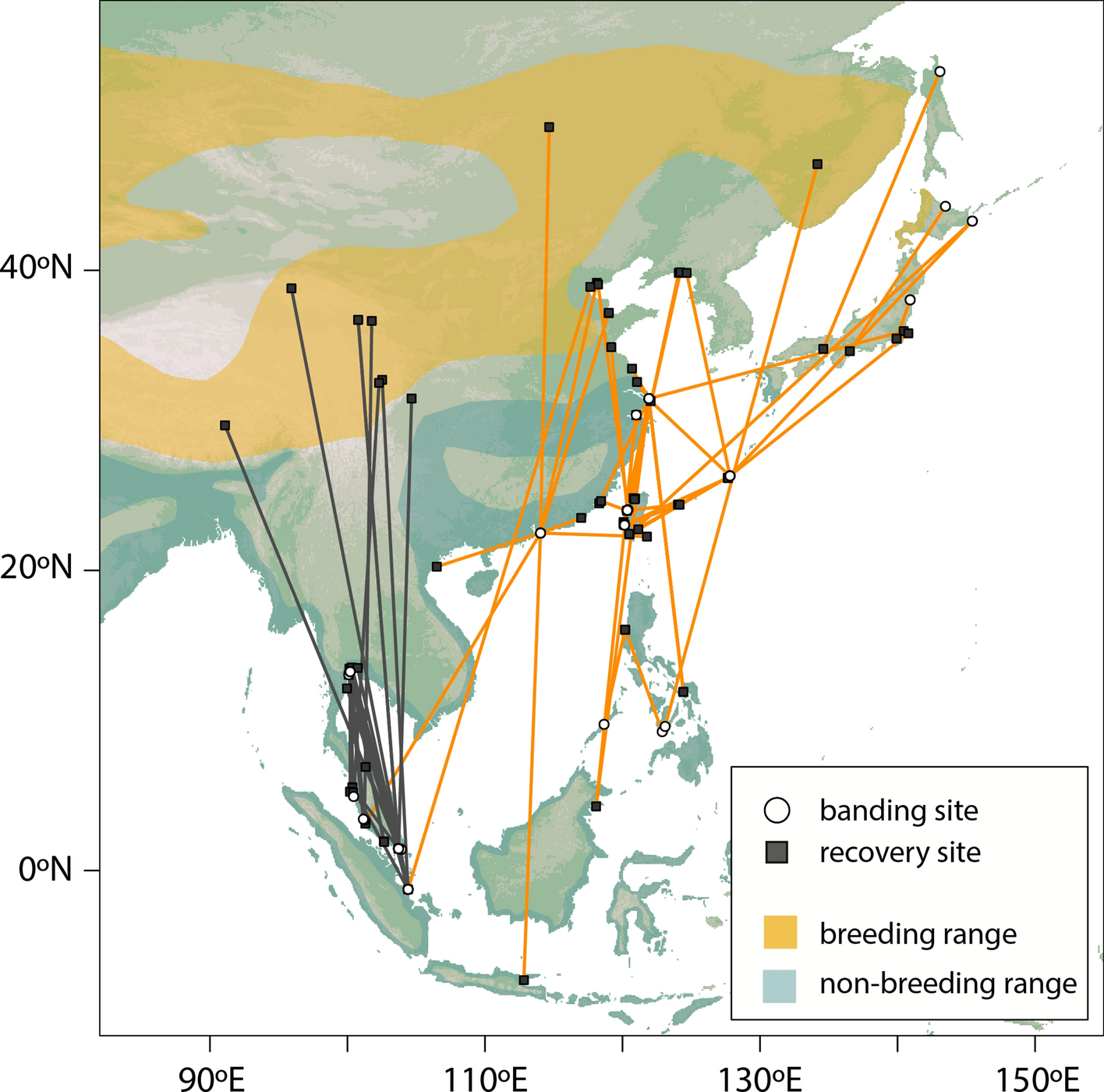This image depicts a detailed map of Asia, resembling a flight grid tracking movement or locations of certain entities. The map displays latitude markers on the left, starting from 40°N at the top and descending to 0°N. Longitude markers at the bottom span from 90°E to 150°E. Within the map, Japan, Korea, China, India, and various Pacific Islands are distinguishable. Colored areas and numerous lines illustrate the data: yellow areas denote the breeding range, blue indicates the non-breeding range, and different shades of green represent landmasses. Orange and black lines, some of which are dotted, connect various points, presumably indicating routes or paths, often intersecting and occasionally forming straight lines between locations. A key in the lower right corner helps interpret these symbols: circles represent banding sites, squares denote recovery sites, yellow squares indicate breeding ranges, and blue squares signify non-breeding ranges. The mainland is mostly green with orange patches, contrasting against a white background, suggesting complex movement patterns across the region.